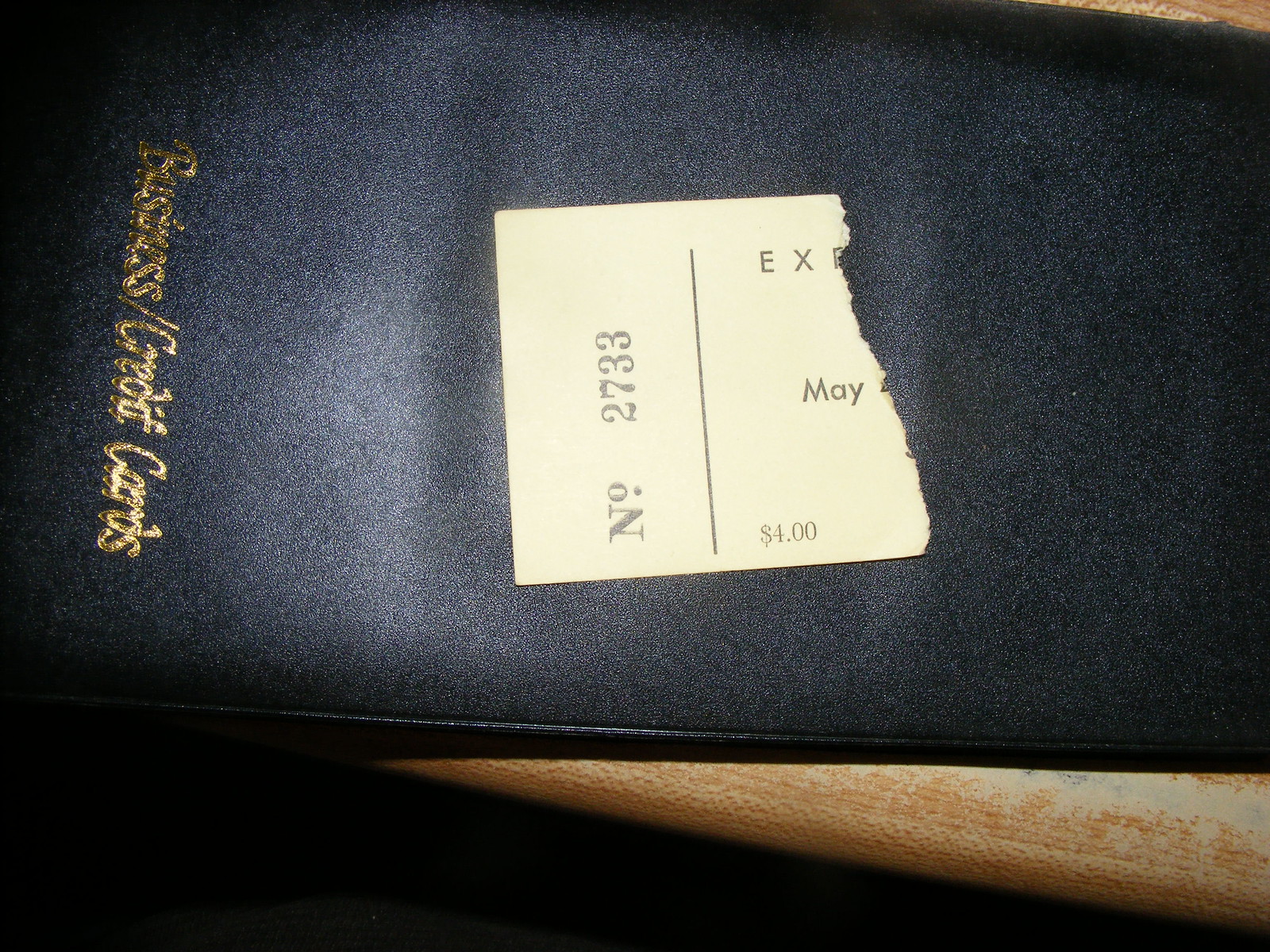In this image, a torn card is prominently displayed on the cover of a black surface that rests atop a table. The bottom of the image features a gray stripe, while the background transitions to black, ending where the table surface begins. The table, characterized by its faded light brown and white hues, supports the black platform. Positioned horizontally across the bottom of the platform is gold text that reads "business credit cards," requiring a rightward tilt of the head to read it properly. The torn card, labeled "NO.2733EXME," displays jagged edges where it has been ripped in half on the right side.